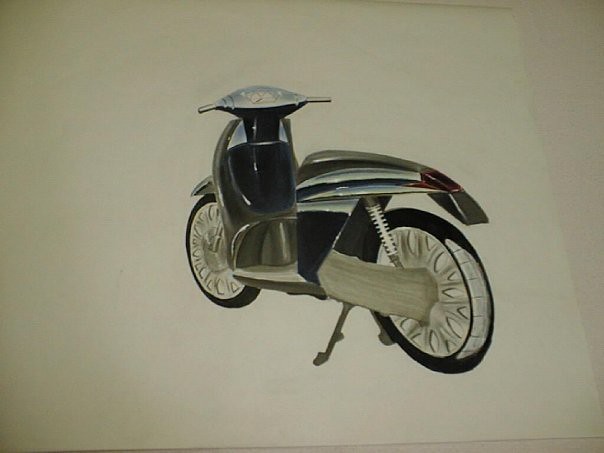This rectangular landscape illustration depicts a motorcycle, rendered with intricate detail. The image appears on a slightly off-white sheet of paper, bordered on the right side and lower right corner by a marginally more white background, revealing a table surface in a subtle off-white shade. The left edge of the paper extends beyond the frame, leaving it unseen.

The motorcycle, angled approximately 45 degrees away from the viewer, positions its rear tire closer and larger in the frame than the front tire, enhancing the perspective effect. Resting on its left-side kickstand, the vehicle's two black tires are complemented by silver-colored spokes. The kickstand itself is gray and visibly protrudes from the side.

The front part of the motorcycle, though partially obscured by the angle, reveals a predominantly black section ahead of the seat area. The handlebars exhibit a flat, elongated oval—resembling the shape of an American football—finished in a silvery hue, with two short silver metal bars extending outward. There are no visible brakes or additional features on these handles, which appear minimalist and straightforward.

The seat of the motorcycle curves gracefully downward at the back, forming a fin-like structure that slopes towards the ground, just above the rear tire. A small red taillight is discernible near the end of this curved fin, adding a touch of color and completing the detailed portrayal of the motorcycle.